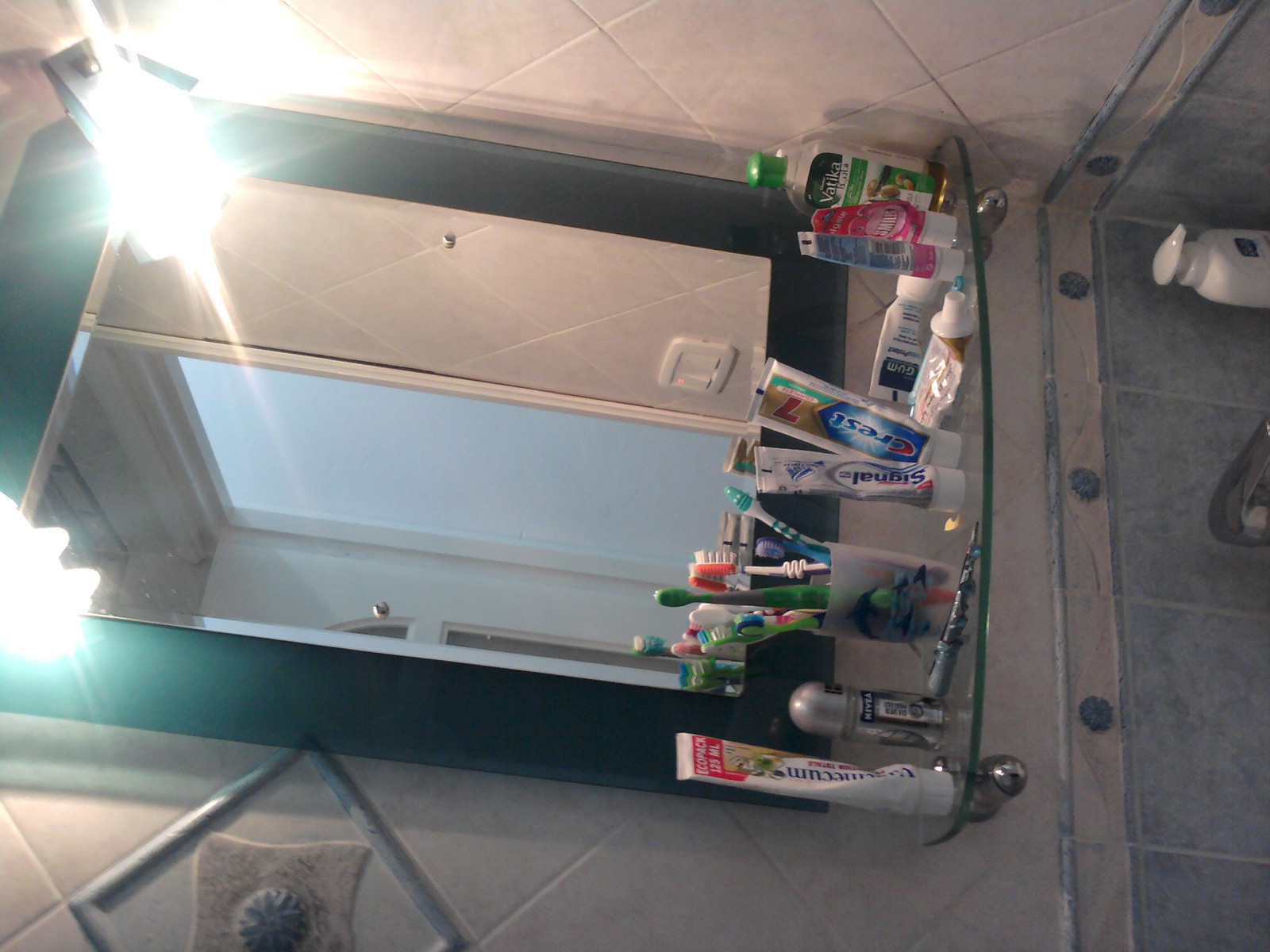This image depicts a contemporary bathroom area above a sink, but the photograph is sideways and should be rotated clockwise. Dominating the scene is a black-framed mirror, which may or may not be a medicine cabinet, flanked by two bright lights in the upper corners. Below the mirror is a clear glass shelf crowded with various toiletries. On the shelf, there's a cup filled with multiple toothbrushes, several different kinds of toothpaste standing on their tops, and some lying on their sides. There is also a silver item, possibly deodorant, and a bottle of mouthwash in one corner. The bathroom features beautiful, intricate tile work with greenish-gray tiles in the lower part and tan tiles with decorative markings creating a trim. The wall also displays some artistic tiles seamlessly integrated among the regular ones. The sink faucet is just visible, accompanied by a white bottle with a pump in the corner. Overall, this bathroom exudes a clean, organized look with some attractive design elements.